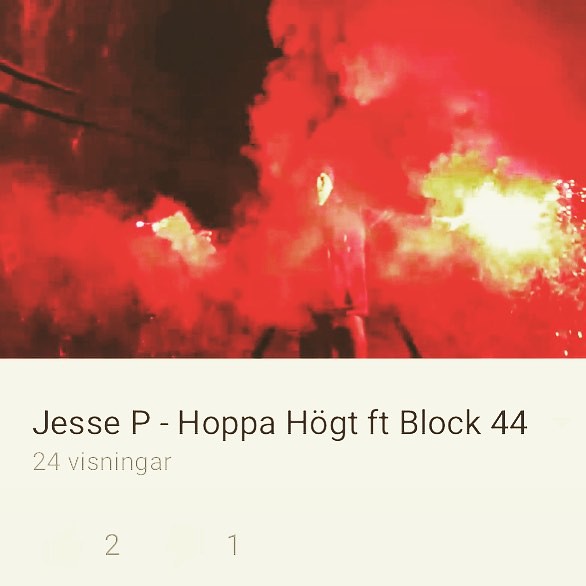The image is a square, colored photograph taken outdoors at night, dominated by dark and reddish hues. It features a person, likely male, wearing a dark jacket and a hat, engulfed in a swirling mass of red smoke, suggestive of flames. The sky forms the black background, with some yellowish areas adding contrast. Below the image, in black and gray text, there is the inscription "Jesse P. Hoppa featuring Block 44." Additionally, it includes the text "24 Visningar" above the numbers "2" and "1" on the bottom left. The overall effect of the image is dramatic, with the person almost obscured by the vibrant and chaotic scene of smoke and color.